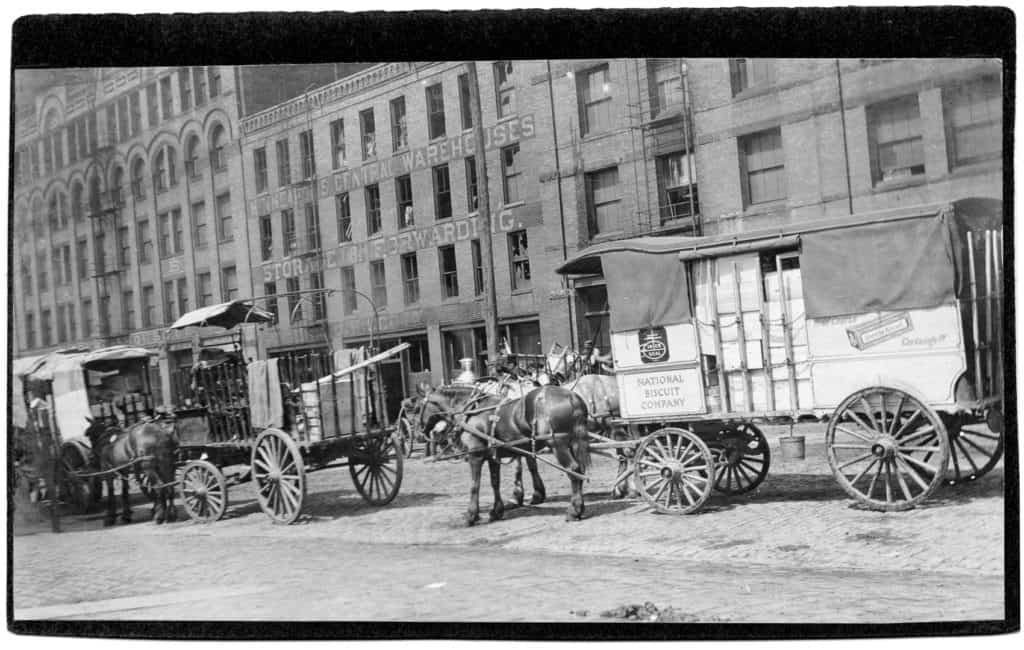This black-and-white vintage photograph, likely taken in the late 1800s, captures a bustling downtown city street. The scene is dominated by several tall, brick multi-story buildings stretching to the top edge of the image. One central building bears a worn sign reading "Central Warehouses, Storage, Forwarding," though the complete text is partially obscured. 

In the foreground, the street is lively with horse-drawn carriages. Most prominent among them, on the bottom right of the image, is a light-colored carriage with a canvas cover and four wooden wheels—two smaller at the front and two larger at the back. This carriage is marked with a sign for the "National Biscuit Company" and is drawn by two horses. There are at least two additional carriages further along the street, their exact details blurred by the photograph’s age. The street exudes an atmosphere of early urban activity, with possible vendors or other street objects visible indistinctly in the background. The entire image is bordered in black, emphasizing its vintage realism.